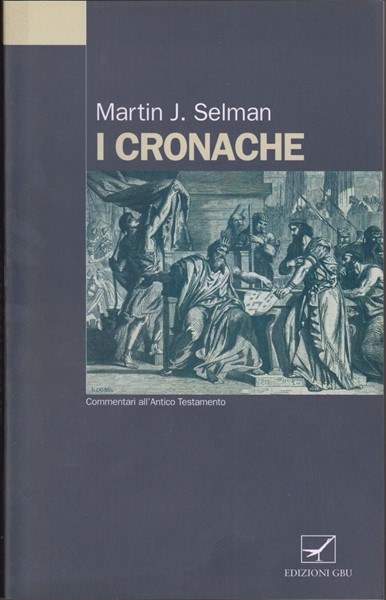This is a detailed description of the cover of a hardcover book titled "I, Cronaci" by Martin J. Selman. The book cover is predominantly a dark purple or black color and is taller than it is wide. In the upper left corner, there is a cream-colored rectangle from which a faint vertical line extends downward to an intricate line drawing.

The drawing depicts an ancient scene, possibly Greek, Babylonian, or biblical, featuring a ruler seated on a throne with his arm outstretched towards a scribe who is holding an unrolled scroll. Surrounding them are multiple individuals, some positioned behind the throne and the scribe, set against a backdrop of columns and pillars. The title of the book, "I, Cronaci," is written in cream-colored capital letters above the image, while the author's name, Martin J. Selman, is displayed in white lettering above the title. In the bottom right corner, there is a logo or name, "Edizone GBU," potentially indicating the publishing company.